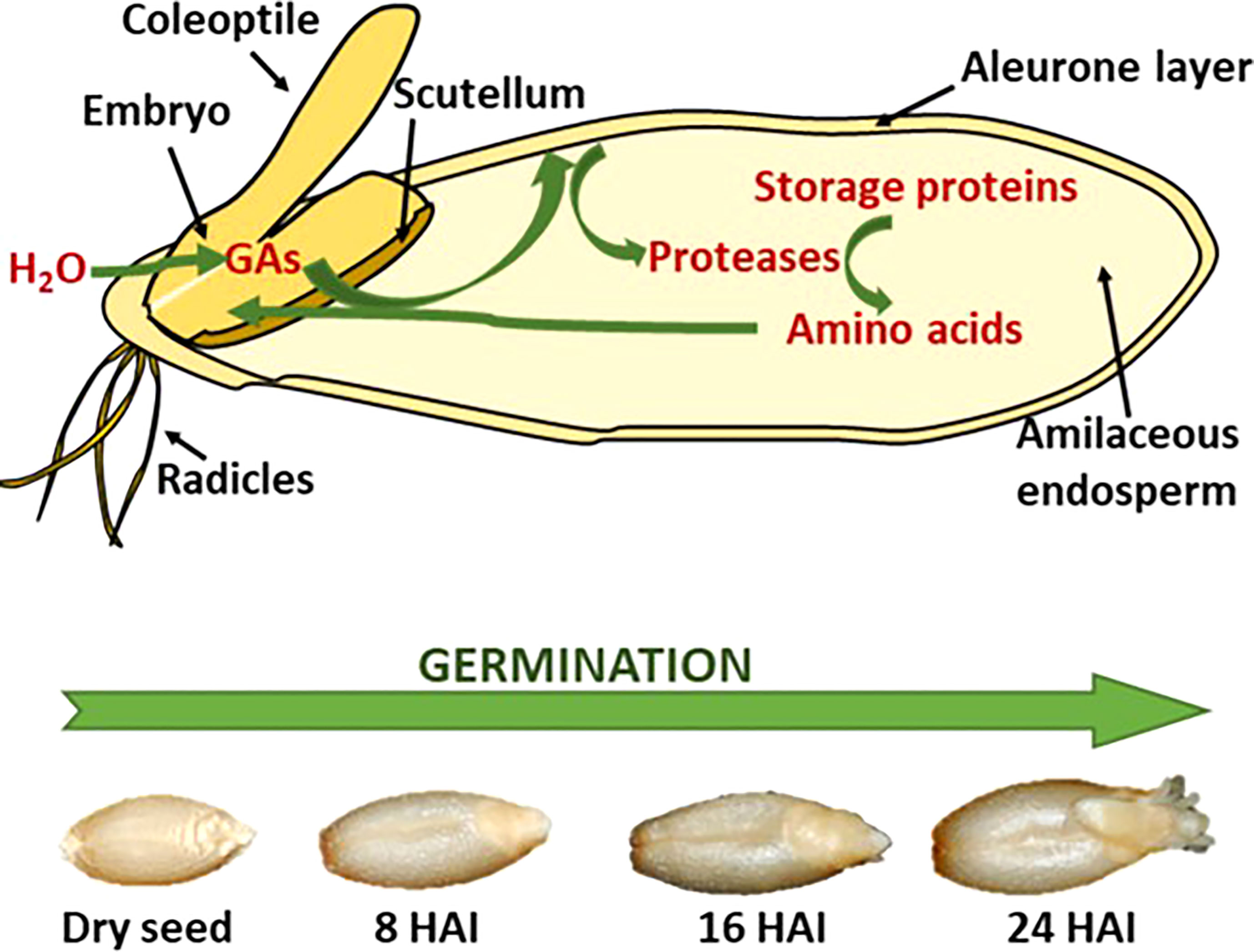This detailed diagram, reminiscent of a biology textbook, illustrates the stages of seed germination. Across the bottom, a green arrow labeled "GERMINATION" points right, indicating the progression of development. Below this arrow, four images depict the sequential stages of a seed transitioning from a dry state, through 8, 16, and finally 24 hours after imbibition (HAI). You can observe the seed swelling and splitting at the tip, culminating in sprouting at 24 HAI. Above the arrow, a detailed cross-sectional drawing labels key parts of the seed: radicles, embryo, coleoptile, scutellum, proteases, storage proteins, amino acids, aleurone layer, and a nutritious endosperm. The diagram also illustrates water uptake and gas exchange, essential for germination, providing a comprehensive overview of the process.